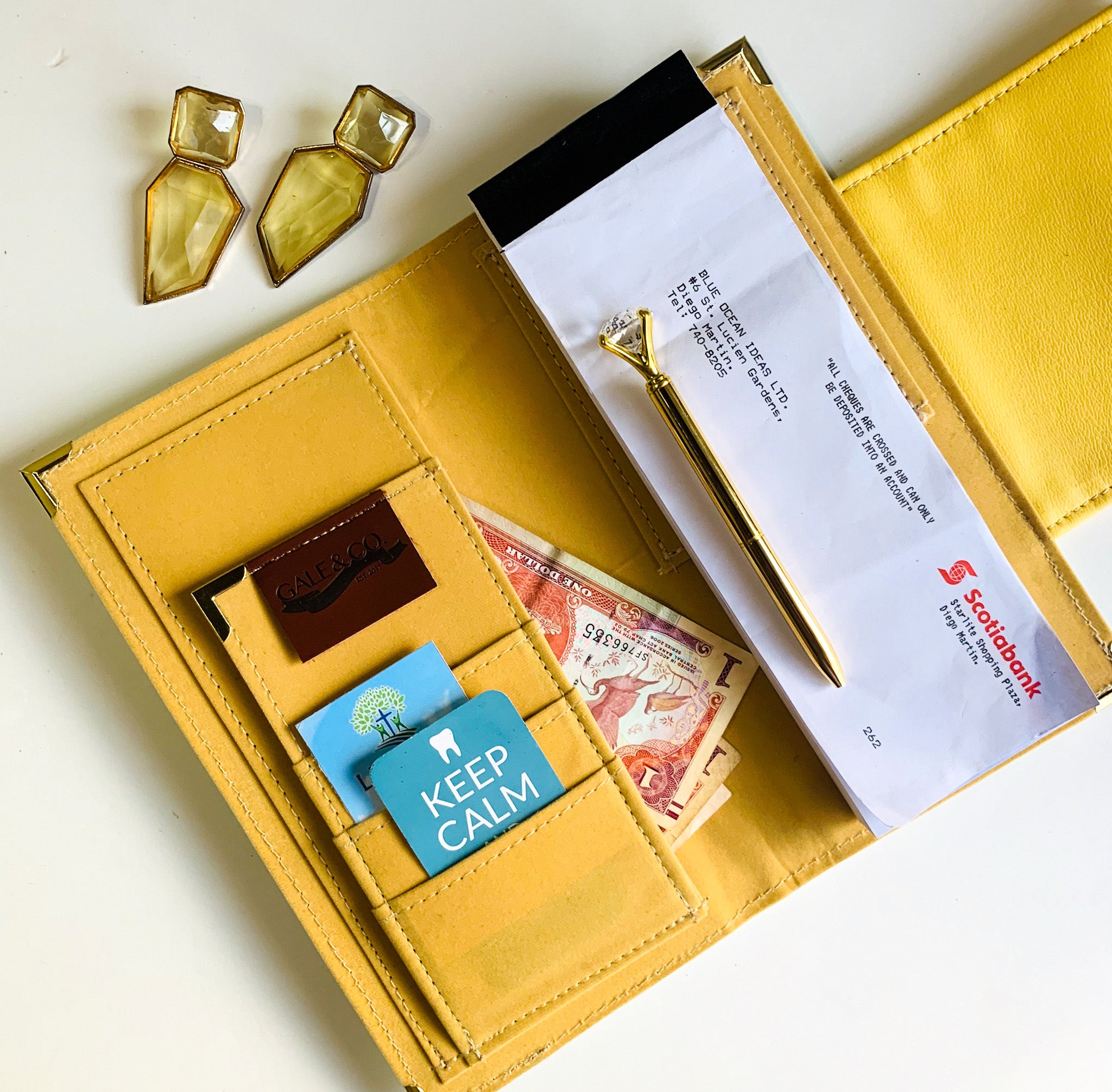The image depicts a vintage mustard-colored leather wallet, displayed on a cream-colored countertop and photographed from a top angle. The wallet is open, revealing various compartments and contents. The interior features several slots for credit cards, including two blue cards, one of which has a drawing of a human tooth with the message "keep calm." A set of European currency notes is visible in one of the larger pockets. The wallet also houses a Scotia Bank checkbook, labeled in red letters and adorned with a border in black. A slender, gold-colored designer pen is attached to the checkbook, which bears the number 262 at the bottom. Additionally, there are amber-colored glass earrings positioned at the top of the wallet. The exterior of the wallet is detailed with metallic triangular embellishments along the edges. Lastly, two green crystals are seen placed on the surface next to the wallet.